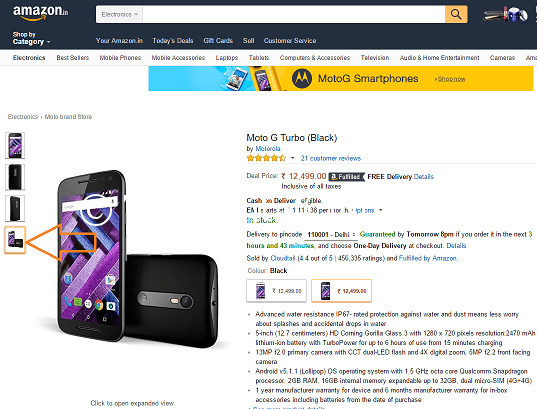This photograph is a screenshot from the Amazon website featuring the Moto G Turbo smartphone by Motorola. The product page displays the camera prominently, along with four different variations of the phone. The Moto G Turbo is showcased in black and has a nearly five-star rating based on 21 customer reviews. The price is listed as ₹12,499, indicating that the currency is in Indian Rupees. The page provides detailed information about delivery options, allowing prospective buyers to make informed choices. Four diagrams illustrate the phone from different angles: the front, the side, the back, and its dimensions. The screenshot only captures the initial section of the product page, offering a glimpse of the product description and other relevant details.